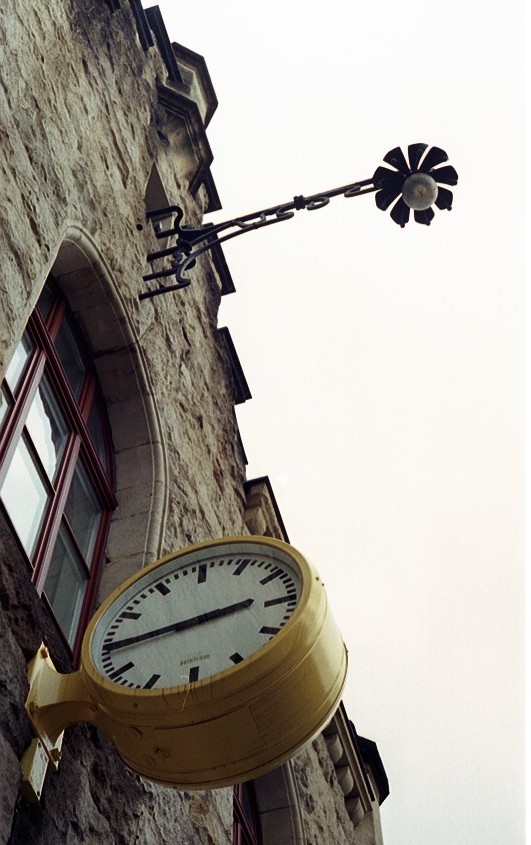This color photograph, taken from ground level, captures the facade of an old building with rough stone brick construction. The angle of the shot looks vertically upward towards an overcast, solid light gray sky, adding a vintage patina to the image's overall composition and coloring. Dominating the center of the image is an arched window framed in red, accentuating the building's old-world charm. Just below this window, a yellow metal clock with a cylindrical shape juts out from the wall, mounted securely with four bolts. The clock's white face features black minute markers arranged without numbers. Above the arched window, there is a fan-shaped weather vane made of black steel, resembling an upside-down flower with a clear light bulb pointing downward from its center. The architectural details and composition suggest a European, possibly English, setting for this beautifully captured exterior.